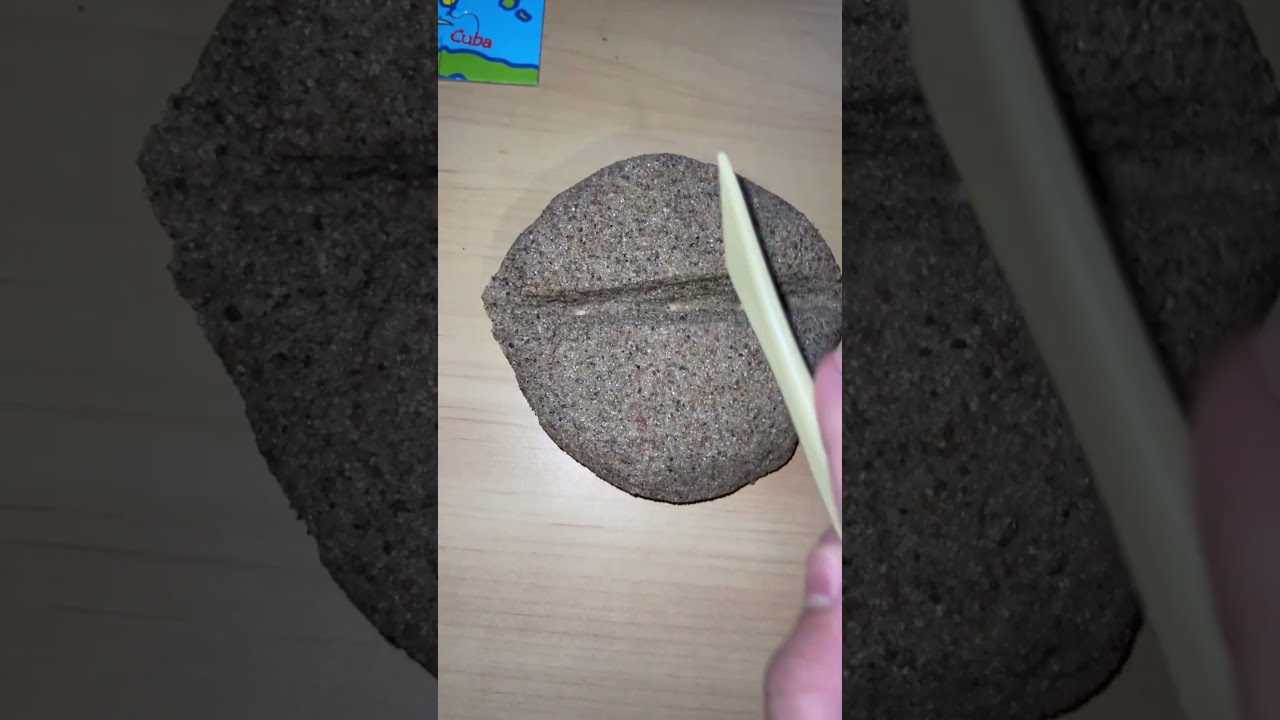The image, taken from a cell phone and formatted in a vertical style, showcases a detailed scene centered on what appears to be a circular, gray, speckled rock or clay-like object resting on a light brown wooden surface. The object has a grainy texture and a noticeable horizontal valley running through its center. A partially visible hand of a Caucasian person, appearing from the bottom right, holds a green plastic artist scraper pressed against the disk, seemingly in the process of modifying or cutting the material. In the upper left corner of the image, a small cartoon map featuring bright blue and green hues and labeled "Cuba" in red letters adds a splash of color. The image is further framed by zoomed-in, faded versions of itself on either side.